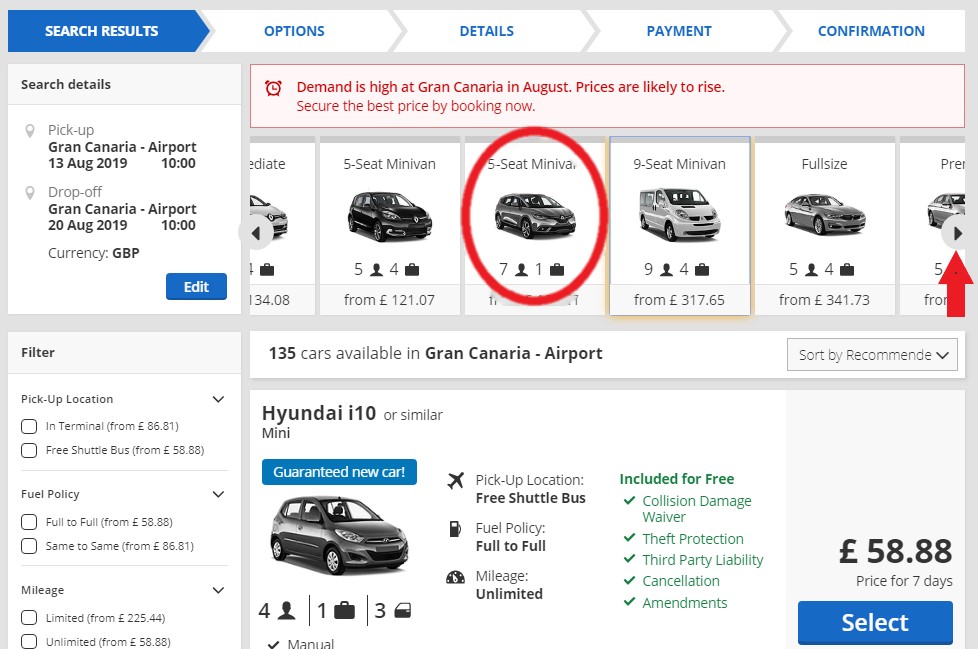This screenshot captures a search results page from an unidentified car rental website. The absence of the company's name, header graphics, and footer graphics leaves the provider anonymous. 

At the top left, within a blue rectangle with white text, it reads "Search Results." Adjacent to this, in blue font against a white background, are the navigation options: "Options," "Details," "Payment," and "Confirmation." A sidebar on the left is labeled "Search Details," showing specifics: "Pickup: Gran Canaria Airport, 13 August 2019, 10:00 AM" and "Drop-off: Gran Canaria Airport, 20 August 2019, 10:00 AM." The currency is listed as GBP (Great British Pounds Sterling). An edit button in blue is located at the bottom right of this section.

Prominently displayed above the search results is a pink banner with red text cautioning, "Demand is high at Gran Canaria in August. Prices are likely to rise. Secure the best price by booking now."

The top row showcases various minivans against a white background, with the selected minivan highlighted by an egg-shaped red oval. Further down, a different listing is shown for a "Hyundai i10 or similar," which guarantees a new car. Accompanying this listing is an image of the car and the price, 58.88 GBP. Below the price, a rectangular blue button with white text reads "Select."